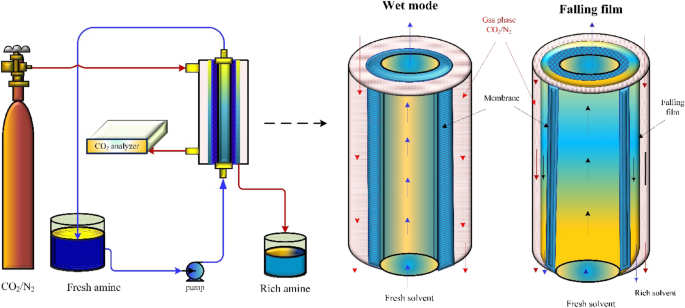The image illustrates a detailed scientific diagram, likely from a textbook, showcasing a contraption involving carbon dioxide (CO2) and nitrogen (N2). Central to the diagram is an orange distributor tank situated on the left, which serves as a reservoir. At the bottom, the diagram labels CO2 and N2, indicating their starting points. From there, the process flows to a CO2 analyzer, a fresh amine pump, and then to a rich amine section. 

Two cylindrical tanks are depicted on the right, one displaying a 'wet mode' and the other labeled 'falling film', both indicative of different stages or conditions within the process. These components and stages are connected through various lines representing the flow of gases and liquids. The diagram uses a color scheme dominated by dark blue, light blue, and yellowish tones, with text annotating important elements such as 'fresh solvent', 'membrane gas phase', and 'rich solvent'.

In addition, there are smaller canister-like figures, one in bronze, connected intricately to the pumps and other components. These elements are also marked with signs like a plus symbol and color-coded parts, further detailing the functional aspects of the system.